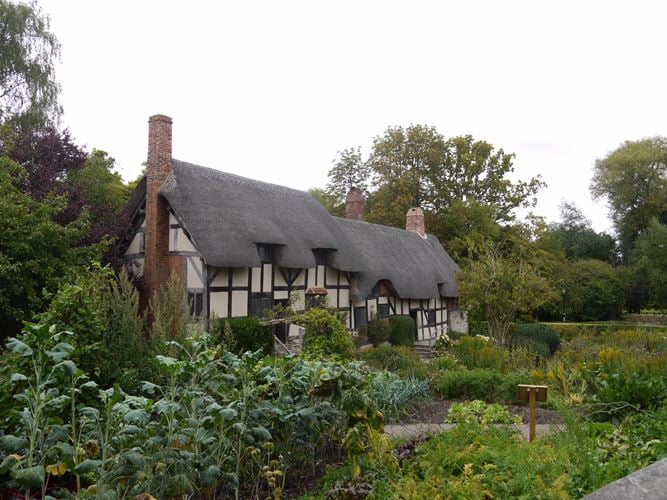The image depicts an outdoor setting featuring a large garden brimming with various shades of green plants and trees. In the lower left corner, dark green leafy plants are prominently displayed, with shorter, lighter green plants to their right. A small wooden sign sits beside these plants, adjacent to a lighter-colored pathway. On the opposite side of the pathway, a different variety of plants flourish alongside some small trees and an array of shrubs in different green hues.

Dominating the center of the photo is an old Dutch-style house with white walls accented by black boards. The dark gray roof, punctuated by brick chimneys and other structural elements, adds to the architectural charm. The surrounding area is lush, filled with tall plants, shrubs, and scattered trees, further enhancing the garden's verdant ambiance. The scene is bathed in daylight, indicating the photo was taken during the day, under a white, clear sky. The overall impression is one of serene, well-kept natural beauty complemented by the stately home.